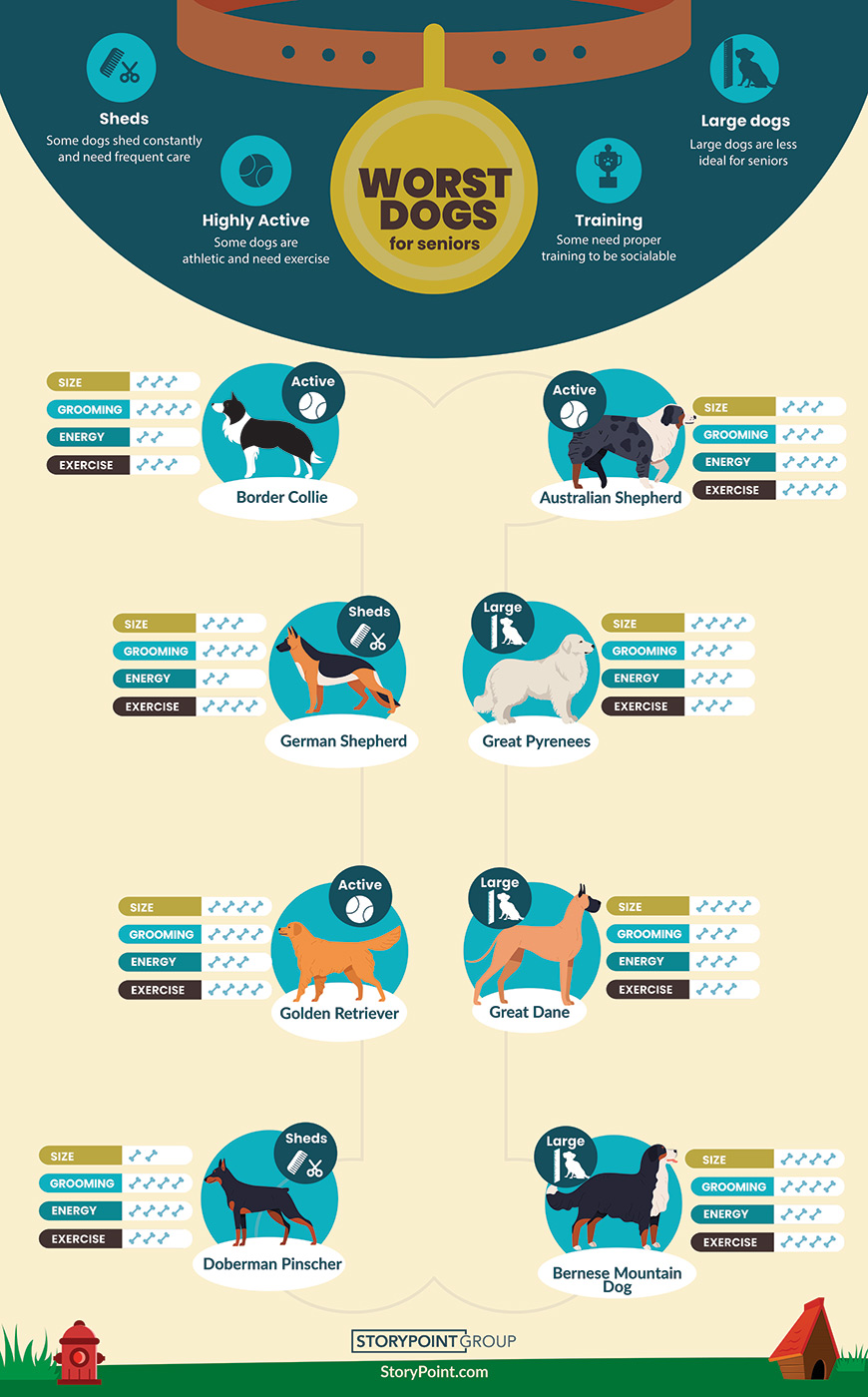The image is a computer-generated diagram, likely from a brochure or magazine, titled "Worst Dogs for Seniors." At the top, there is a blue spot featuring a brown dog collar with a gold dog tag that reads "Worst Dogs for Seniors" in brown letters. Surrounding this are circles with the words "Highly Active," "Training," and "Large Dogs." Below, on a white background, there are illustrations of eight dog breeds identified as unsuitable for seniors: Border Collie, Australian Shepherd, German Shepherd, Great Pyrenees, Golden Retriever, Great Dane, Doberman Pinscher, and Burmese Mountain Dog. Next to each dog, a bar graph rates them on size, grooming, energy, and exercise needs. At the very bottom, a green banner stretches across the diagram, accented with a drawing of a red fire hydrant on one side and a dog house on the other. This detailed and informative chart appears to be created by StoryPoint.com.